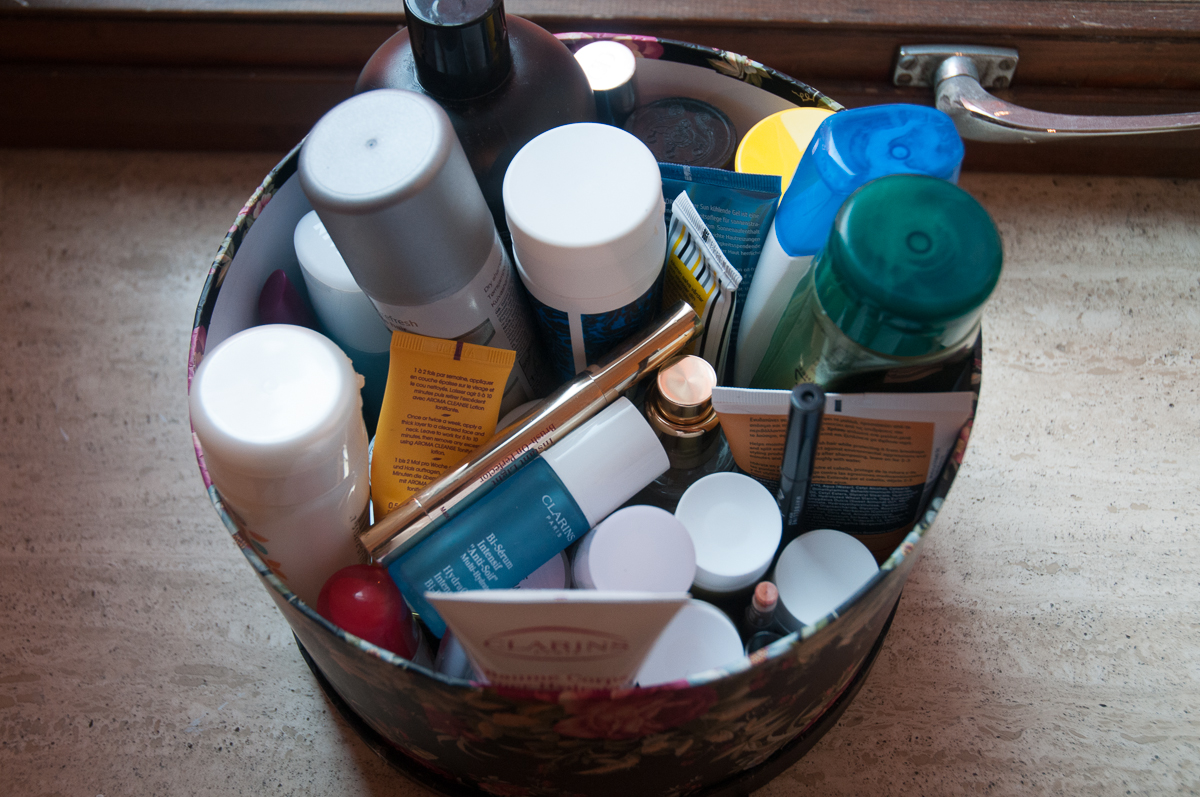The photograph depicts a vintage, circular container adorned with a floral pattern, suggesting it hails from the 1980s or 1990s. The container, seemingly made of cardboard, rests on a wooden surface and occupies the foreground. Behind it, a wooden window frame is visible, complete with a metal handle positioned to the right.

Inside the container, a variety of products are tightly packed, primarily consisting of healthcare and beauty items. Although many labels are not fully visible, some appear to begin with the letter "C," possibly hinting at brands like Clarins. The assortment includes items that resemble hairsprays, moisturizers, and potentially spray paints. Notably, a large black bottle, likely a hair dye, conditioner, or shampoo, stands at the back of the container. The image offers a nostalgic glimpse into a collection of personal care products densely packed within an old-fashioned container.